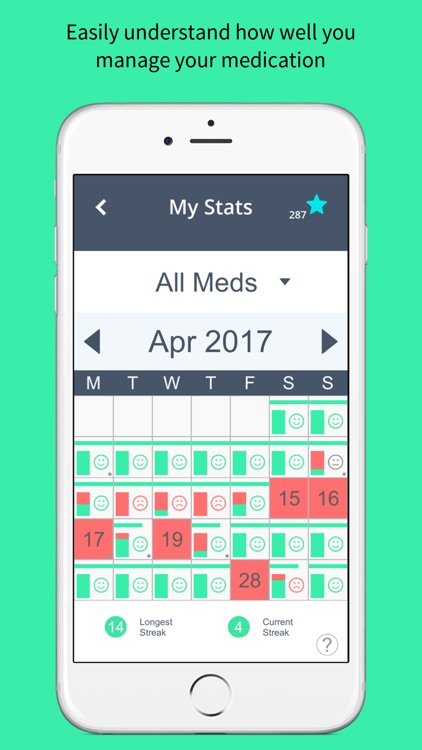This is a detailed and descriptive caption of the product feature photo:

The image is a screenshot showcasing a product feature, specifically a medication management app displayed on a white iPhone. The background of the image is a light green shade, which sets a calm and soothing tone. 

At the top of the image, a bold black font headline reads: "Easily understand how well you manage your medication." Below this, prominently in the center, there is a large image of a white iPhone, displaying the app interface clearly. The iPhone's buttons on the left and right are visible, grounding the image in the recognizable Apple aesthetic.

The app screen is designed with a blue header at the top, featuring the text "My Stats" in large white letters. To the right of this header is a single blue star, with the number "287" in small white text positioned just below and to the left of the star.

The main body of the app screen is white, with the text "All Meds" centered at the top and accompanied by a drop-down box to the right. Below this section, a gray panel displays the text "April 2017" in big blue letters, centered for clear readability. There are triangular icons on the left and right sides of this panel, which are used to scroll through different months.

Below this panel, there is a calendar section starting with a horizontal blue banner featuring the days of the week: Monday, Tuesday, Wednesday, Thursday, Friday, Saturday, and Sunday. The dates within the month are displayed in squares, each containing either a green smiley face or a red frown face. Notably, the numbers 15, 16, 17, 19, and 28 are highlighted with red boxes. 

At the bottom of the screen, on the left side, there is a green number "14" accompanied by the text "Longest streak." On the right side of this section, a green bubble with the number "4" displays the text "Current streak," providing a clear summary of the user’s medication adherence records.

This detailed description captures the visual and functional elements of the product feature photo, highlighting how users can easily track and manage their medication through the app interface.